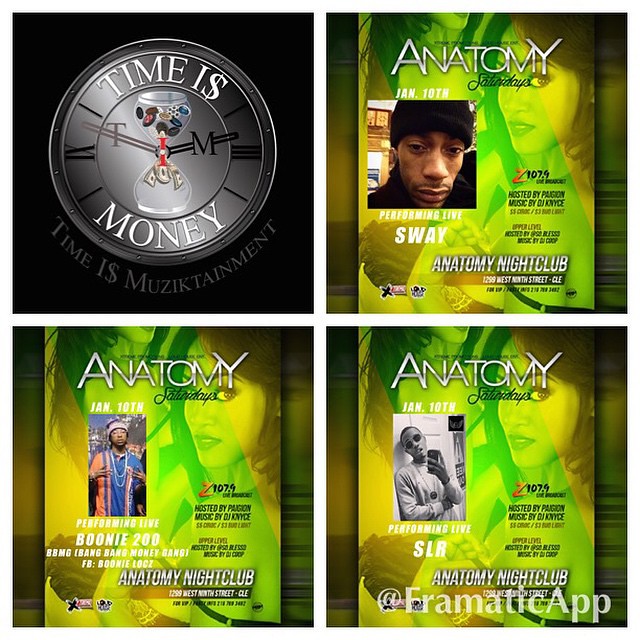This is an image or graphic consisting of four distinct posters arranged in a 2x2 grid. The top left poster features a black background with an intricate overlay of a clock and hourglass. Positioned within the hourglass are poker chips and money instead of sand, with the prominent text: "Time is Money, Time is Musictainment."

The remaining three posters, located in the top right, bottom left, and bottom right, all promote events at Anatomy Nightclub with a consistent green and yellow theme. They are all headline "Anatomy Saturdays" at the top and "Anatomy Nightclub" at the bottom, along with the venue's address: "1299 West 9th Street, CLE."

The top right poster showcases a close-up selfie of a man wearing a black beanie, captioned "Performing Live, Sway" for an event on January 10th. The bottom left poster features a black male artist in an orange and blue hoodie, labeled "Performing Live, Boonie 200, BBMG, Bang Bang Money Gang, FB Boonie Locks." The bottom right poster advertises a performer named SLR, depicted wearing sunglasses and a chain, with his head tilted to the side.

A watermark reading "@from attic app" appears in the lower right corner of the overall graphic. The entire image measures approximately seven inches by seven inches and is of high quality.